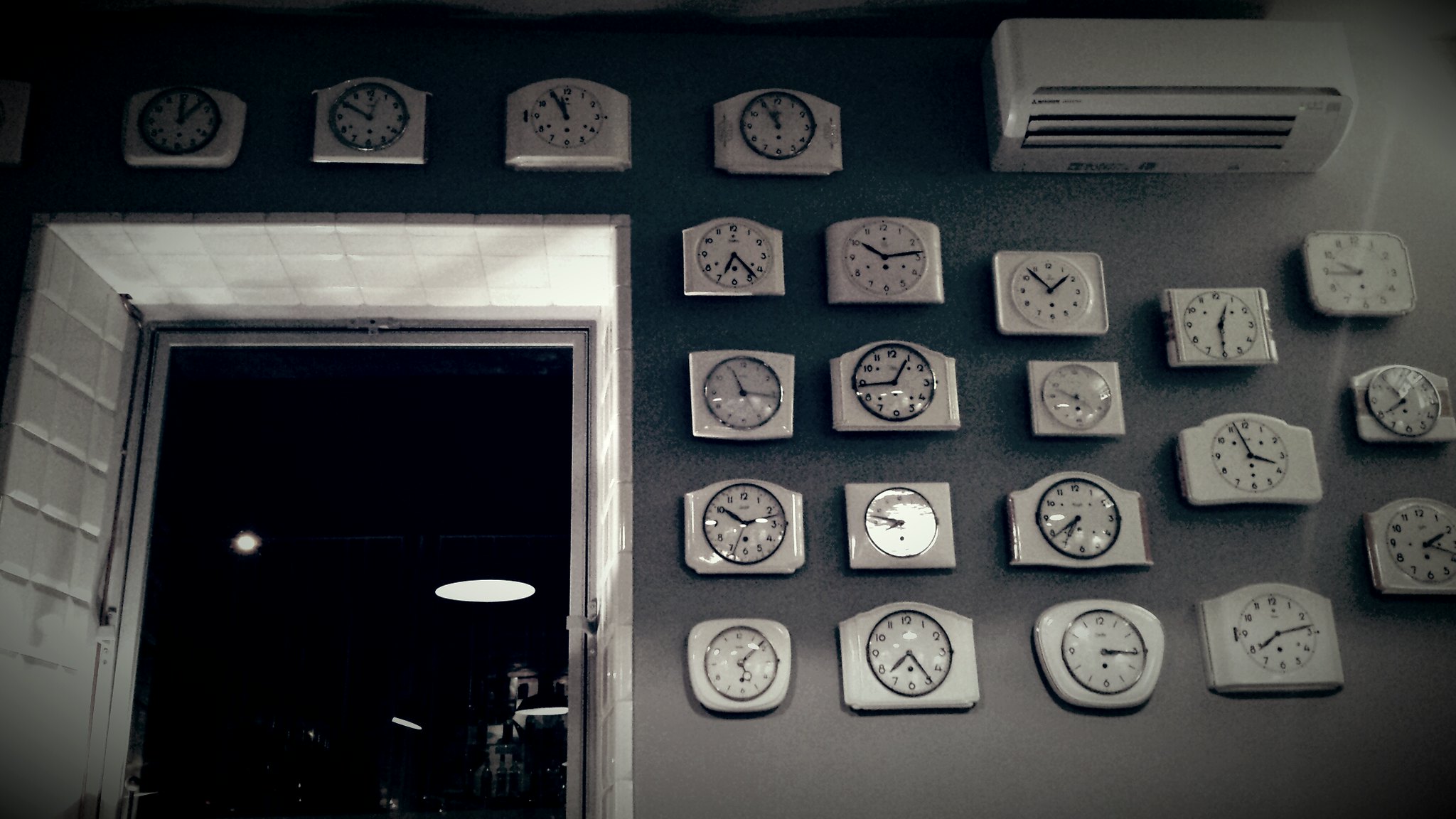This black and white interior photograph showcases a gray wall meticulously adorned with a diverse arrangement of white clocks. These clocks, totaling 19 in count, are set uniformly apart, each displaying different times with black numbers and hands against their white faces. The clocks vary in shape: while many are rectangular, others include rounded edges and curved squares.

In the top right corner of the image, a white, oblong split air conditioning unit, reminiscent of a larger sleek bread box, is affixed to the wall. To the left of the image, there's a distinct doorway bordered with white brick tiles. The interior of the doorway reveals a stark contrast with a deep black background illuminated by a solitary, oval ceiling light, reminiscent of an interrogation scene, adding an eerie ambiance to the overall composition.